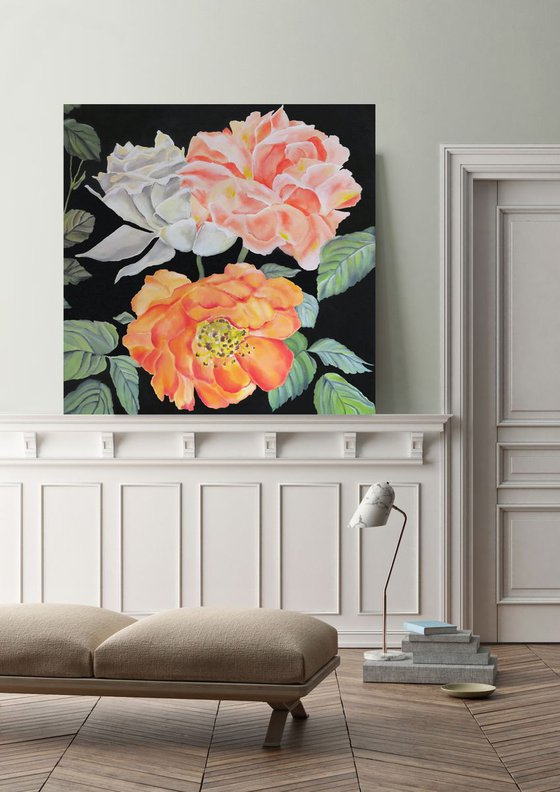This image features a stylish yet minimalistic living room area, likely a stock photo capturing the tastefully designed space of a sophisticated apartment or house. The floor is laid with herringbone-patterned wood slats, providing a distinct and elegant touch. Dominating the scene is the wall, whose bottom half is adorned with white, ornate molding and chair railing, while the upper portion reveals a pale green or creamy lime shade, lending a subtle yet serene color contrast.

To the left of the frame is a low chaise lounge with tan cushions, partially visible as it peeks in. A striking art installation appears towards the center-right consisting of several gray rectangular prisms stacked upon each other, creating a makeshift stand. Atop this stand rests a book and a sleek desk lamp with a white marble base and a bronze stem. Beside the stand, a small dish or ashtray lies on the floor.

The focal point of the room is a captivating painting towards the top left of the image. The painting, set against a dark background, portrays a vivid assortment of roses in varying hues of white, peach, pink, and yellow, accented with lush green foliage. This oil or acrylic artwork adds a burst of color and life to the otherwise muted room. A partially visible, ornate white door is present on the right, enhancing the classic yet modern aesthetic of the space.